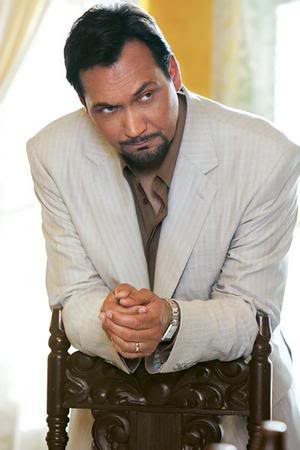The photograph features a man leaning on the back of a solid dark brown wooden chair, his elbows resting on its top. His hands are clasped together towards the front. His face, adorned with a goatee, is turned slightly to the right, capturing a severe and skeptical expression, while his body faces frontwards. He is dressed in a light grey business suit, paired with a light brown button-up shirt that has the top three buttons undone, and matching light grey pants. A silver wristwatch with a square head adorns his right wrist, and a gold ring graces his ring finger. The background reveals a yellow wall with two windows, through which daylight streams in, illuminating the room. Each window features drawn curtains, enhancing the light ambiance of the interior space. The chair he leans on is ornate, showcasing a leaf pattern on its sides and top.